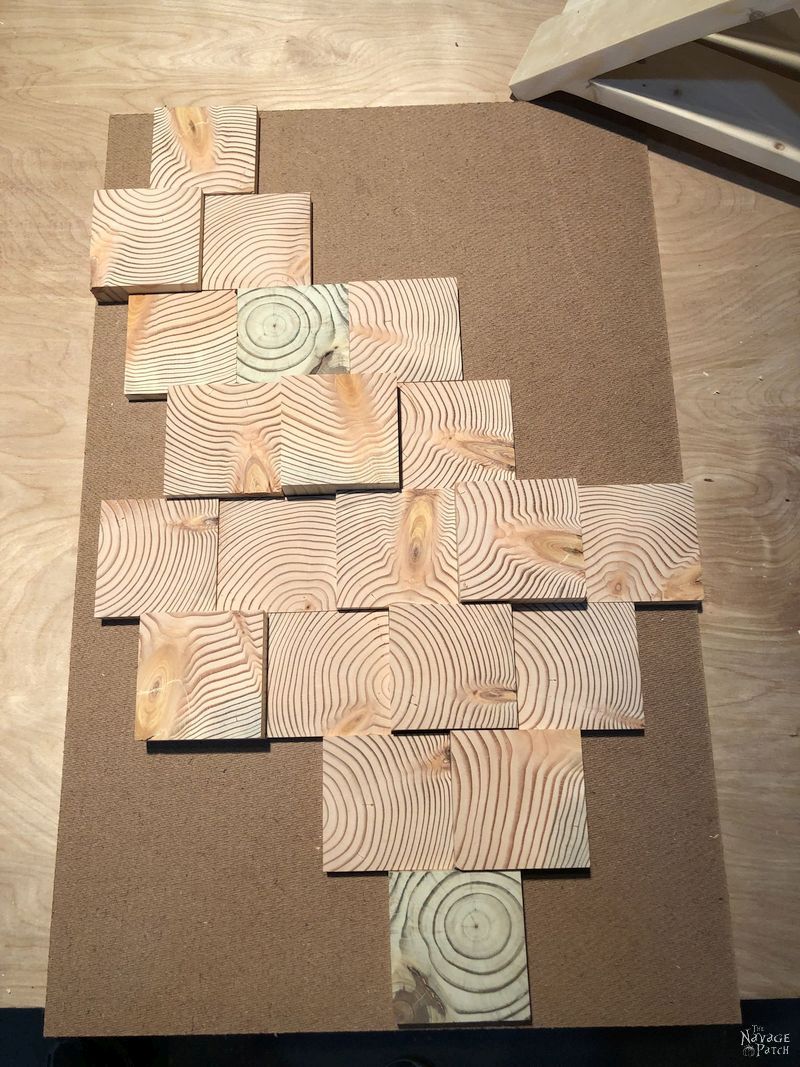The image depicts a collection of approximately twenty thinly cut wooden squares, each displaying unique wood grain patterns. These wooden tiles are arranged on a light brown, particle board surface that resembles a very light shade of beige wood. Positioned in an intricate pattern on the left side of the table, the tiles create a design where the number of tiles in each row varies, ranging from one to five squares. In the top right corner of the photograph, part of a wooden table leg is visible. The bottom right corner of the image features the text "The Navage Patch" in a distinctive, funky-style font. This detailed arrangement captures the natural beauty and distinct texture of each wooden piece, with their swirled, wavy designs reminiscent of onion cuts.